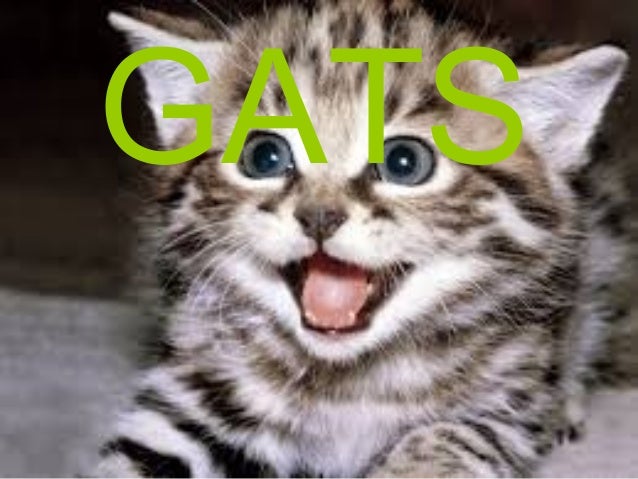The photograph captures a juvenile gray tabby kitten with distinctive black stripes and white spots, lying on a gray fabric carpet. The kitten's face is the main focus, showing off its white-muzzled mouth that is partially open to reveal a bright pink tongue. Its gray eyes with black irises are looking up to the right, and its triangular, pointed ears are white on the inside and tan on the outside. The background is softly out of focus with indistinct shadows, adding depth to the image. Adding a modern twist, the word "GATS" appears in vivid green letters overlaying the kitten's face, blending photographic realism with typographic elements. The overall image, though slightly blurry, evokes a playful yet serene atmosphere, presenting the kitten in a moment of relaxed curiosity.